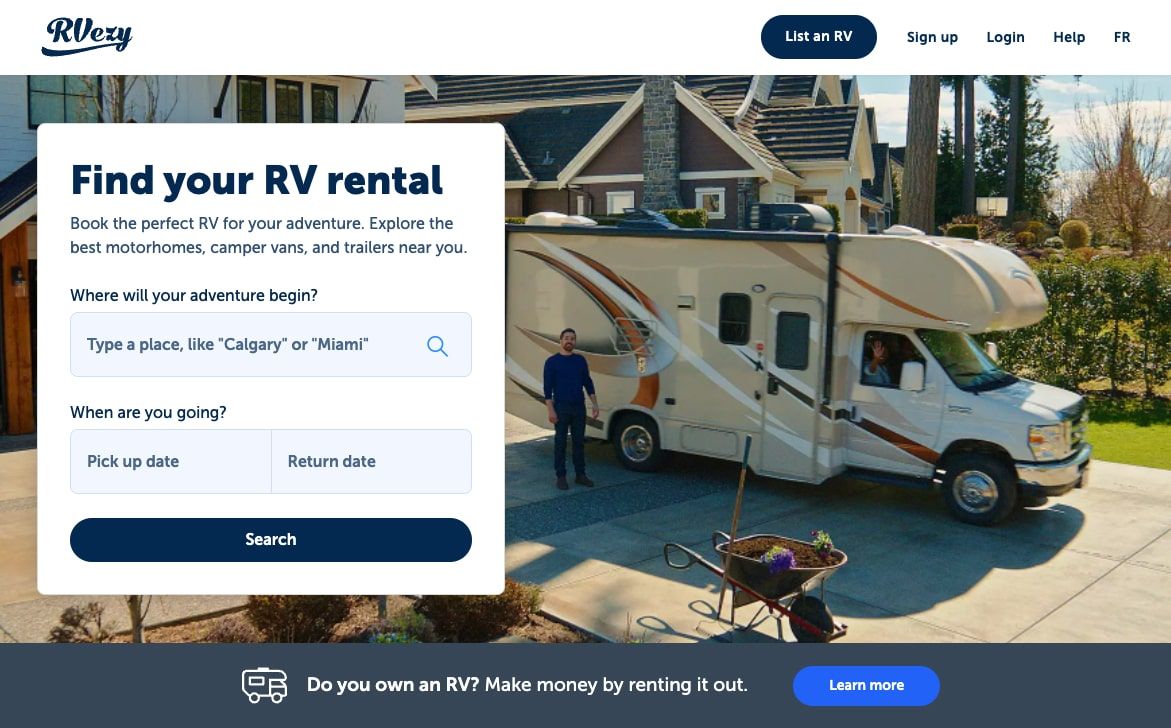This is a webpage belonging to RVZ (spelled R-V-E-Z-Y), a company that specializes in renting RVs. The logo, which is simply the name RVZ, is prominently displayed in the upper left-hand corner of the page. On the far right side of the header, there are five drop-down menus offering various features: a list of available RVs for rent, a sign-up option for new members, a login feature for existing members, a help menu, and a menu labeled "FR," the purpose of which is unclear.

Dominating the page is an expansive image showing a man standing outside of an RV, likely one he has just rented. The RV appears to be parked at his house, and there's another person visible in the front passenger seat, suggesting they are preparing for a trip. Overlaying this scene is a white search box with blue and black text, where users can enter their desired rental location, pick-up date, and return date, followed by a search button to look up available RVs.